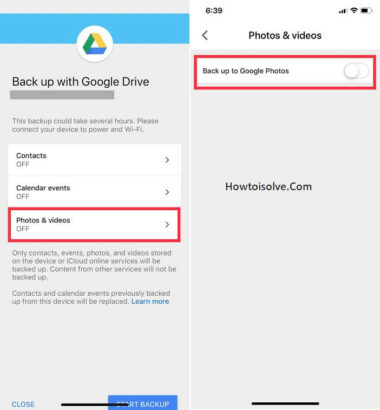Certainly! Here is a detailed and descriptive caption based on the provided voice caption:

---

The image comprises two distinct sections side by side. The left section displays the "Backup with Google Drive" interface. Here, a progress bar in grey runs approximately three-quarters across, indicating the advancement of the backup process. A warning message below the bar reads, "This backup could fail. Please connect your device to power and Wi-Fi." Additionally, toggles for Contacts and Calendar Events are switched off, and options for Photos and Videos display a status of 'off'. At the bottom, there are two interactive buttons: a blue "Close" button on the left and a "Start Backup" button on the right.

In the right section, the interface is dedicated to "Photos and Videos". A highlighted bar, outlined in red, marks the "Backup Google Photos" option. Below this section, a reference to the website "howtoisolve.com" is visible. This part of the image also emphasizes steps to manage the backup of photos and videos from the device.

---

This detailed caption includes all necessary elements to understand the content and functionality shown in both sections of the image.